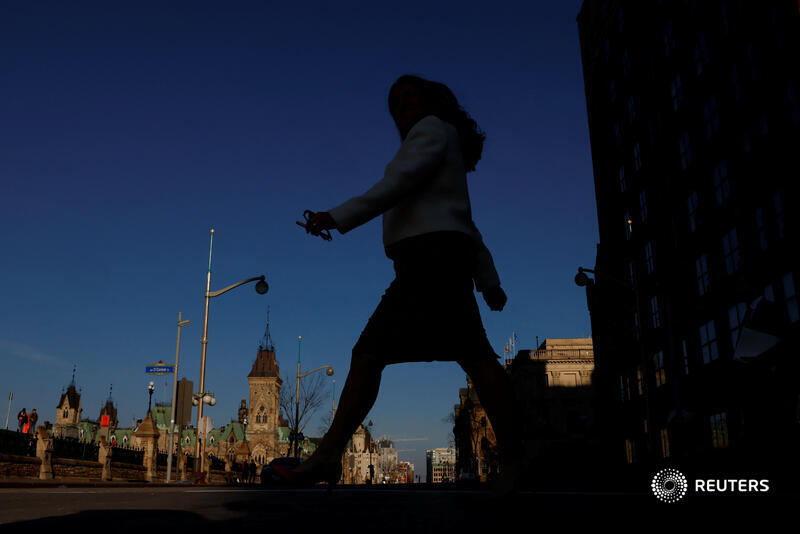This high-contrast, horizontally aligned rectangular photograph captures an early evening scene dominated by a dark blue sky, which spans the majority of the middle and upper left sections of the image. Below this vibrant sky lies a cityscape with brownstone buildings, several with green roofs, and one prominently featuring a steeple. A strikingly dark area on the far right hints at a taller building, though it's barely visible aside from a few windows due to the darkness. Central to the photograph is the silhouette of a woman, depicted striding confidently from right to left, her long hair and knee-length skirt defining her shadowy form. She appears to be holding a pair of sunglasses in her left hand, her arms swinging with her notable stride. The vantage point from the ground up makes her appear imposing against the distant, smaller buildings and light posts. Notably, in the lower right-hand corner, there is a white circular logo with the word "Reuters" inscribed beside it.